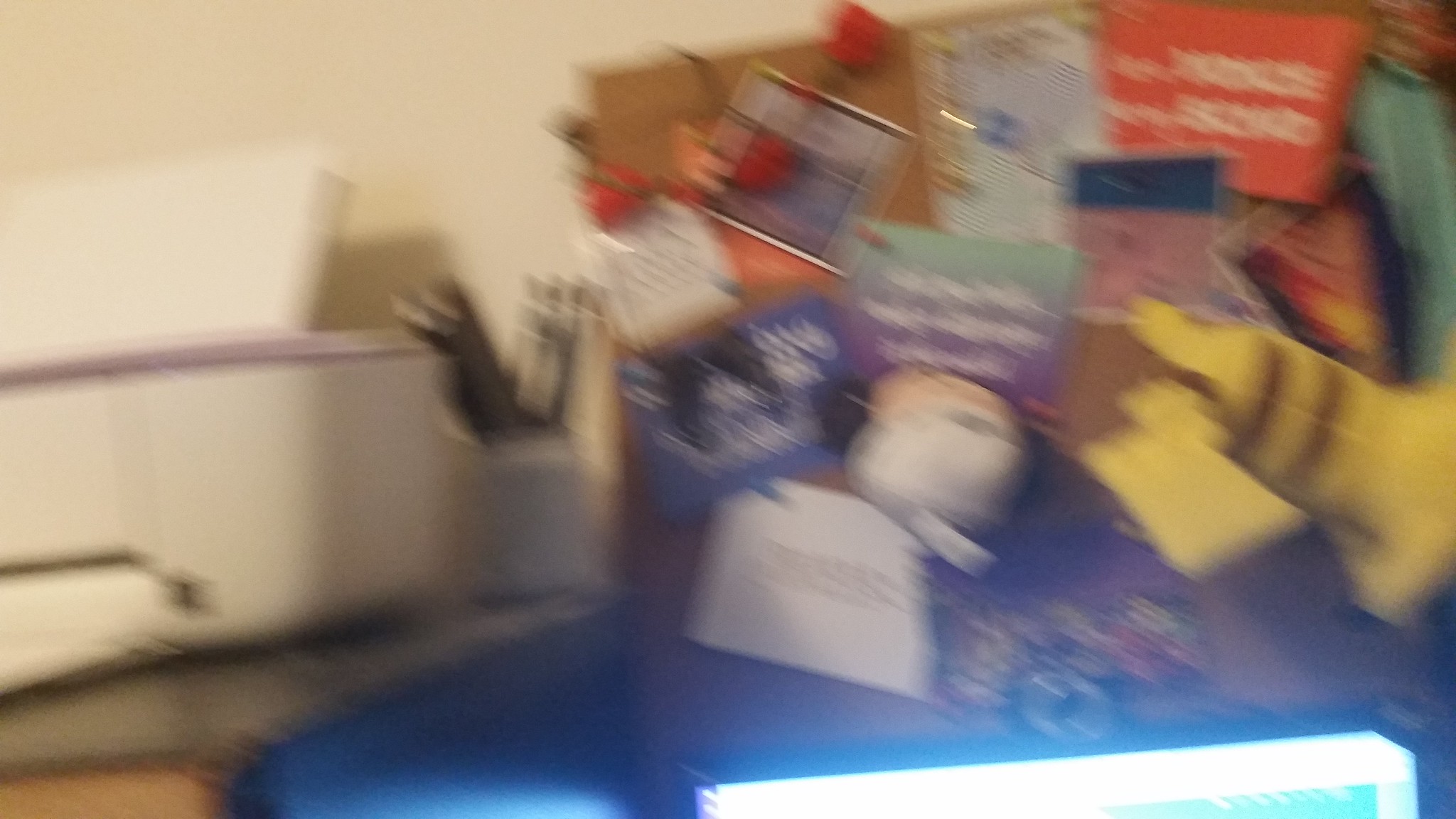A blurry image captures the essence of a home office setup. Despite the lack of sharpness, several key elements are discernible. Positioned at the bottom is a glowing, bright light indicating the presence of a thin laptop, possibly used for work or study. To the left of the laptop sits a table adorned with an HP printer, essential for printing documents and resources. On the right side of the office space, a cluttered cork board draws the eye. This board is adorned with various items, including postcards or greeting cards, which may feature inspirational quotes. Prominently displayed among these items is a Pikachu character from Pokemon, adding a playful touch to the otherwise functional space.